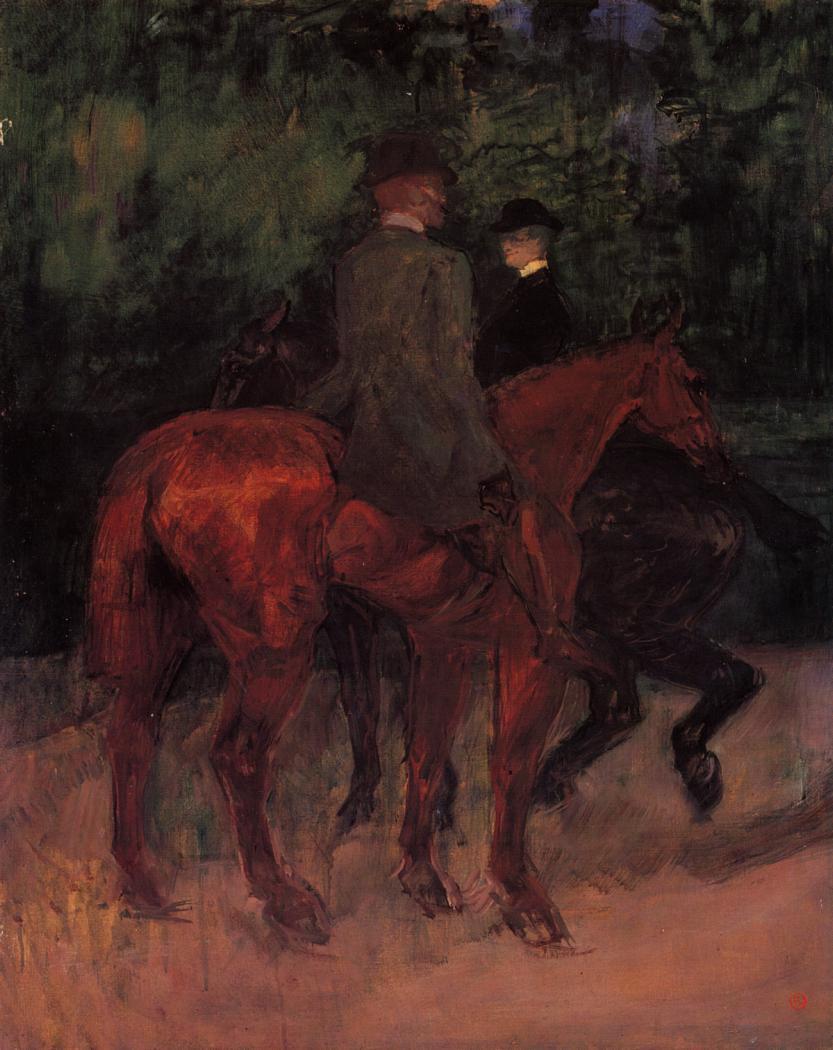This color oil painting titled "Man and Woman Riding Through the Woods," created by Toulouse-Lautrec in 1901, features a post-Impressionism, Art Nouveau style. The painting, in portrait orientation, depicts two figures riding horseback against a backdrop of murky, dark greens suggesting a wooded area at dusk. In the foreground, a woman is shown riding a brown horse, wearing a long dark green jacket, a white-collared shirt, and a top hat. Her horse has one of its legs raised as if trotting. Behind her, a man is depicted atop a black horse, wearing a dark overcoat, a black top hat, and a white shirt. His figure is partially seen, facing left, with his back slightly turned to the viewer. The ground beneath the riders is brown dirt, and the brushstrokes convey a detailed, non-abstract representation, though the overall scene is shadowy and dimly lit, adding to the painting’s dark, atmospheric quality.